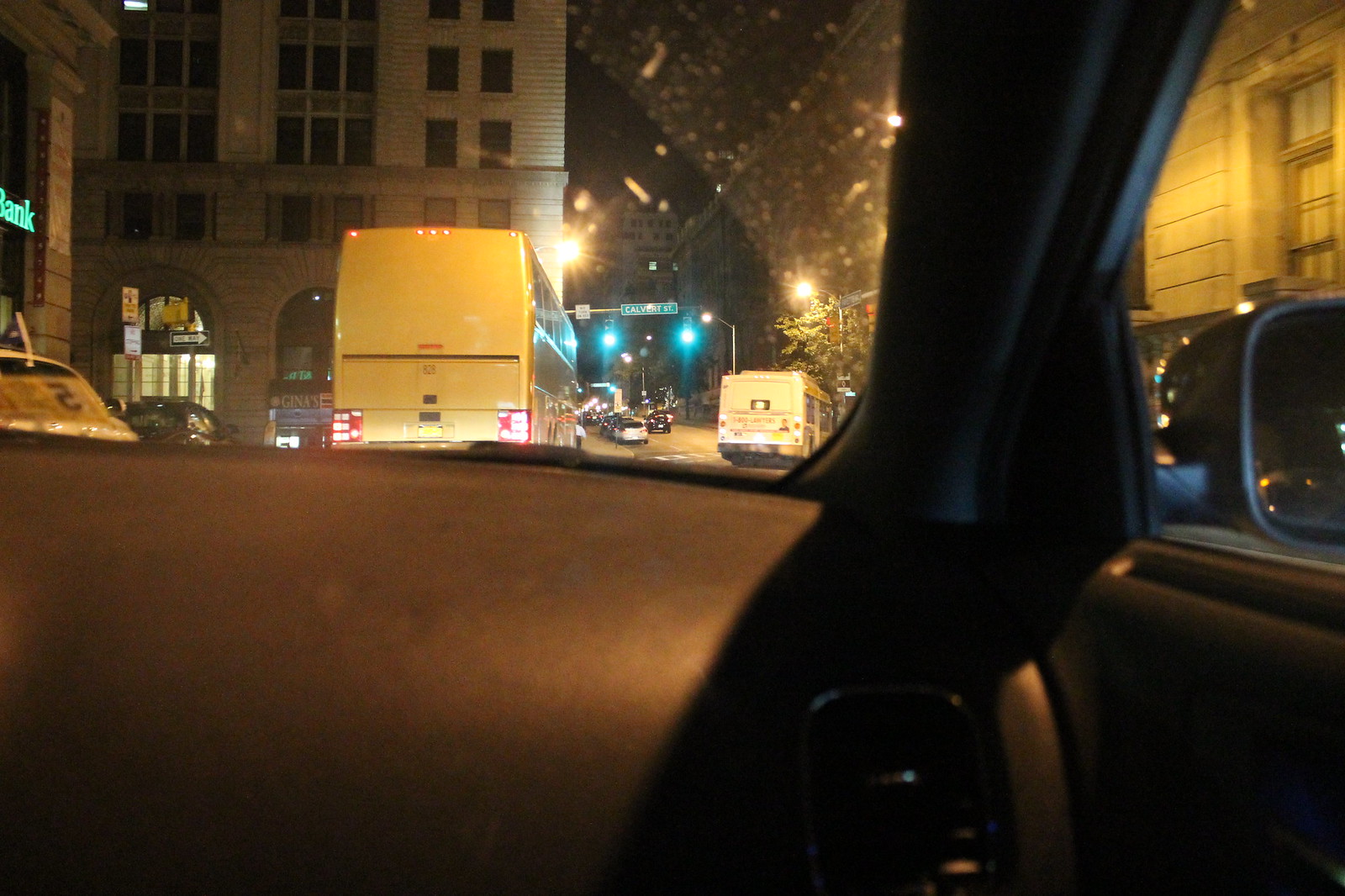In this nighttime image taken from the passenger side of a vehicle, the black dashboard occupies the bottom half of the photo. The car appears to be parked in a downtown area, evident by the tall office buildings with dark windows, indicating they are closed for the night. The dashboard also features a rearview mirror.

Through the car's windshield, the illuminated city reveals several details. Two white vehicles, possibly a cube van and a transit bus, are visible in front of the car, along with other parked cars lining the street. In the distance, green traffic lights are evident, guiding the night traffic. Street signs are partially readable, with one indicating that an upcoming turn would lead to Calvert Street. Additional signage includes "Gina's," possibly a restaurant, and "bank," suggesting the presence of a financial institution. The scene is framed by a mixture of commercial buildings and what appears to be a courthouse, painting a bustling, urban nighttime tableau.